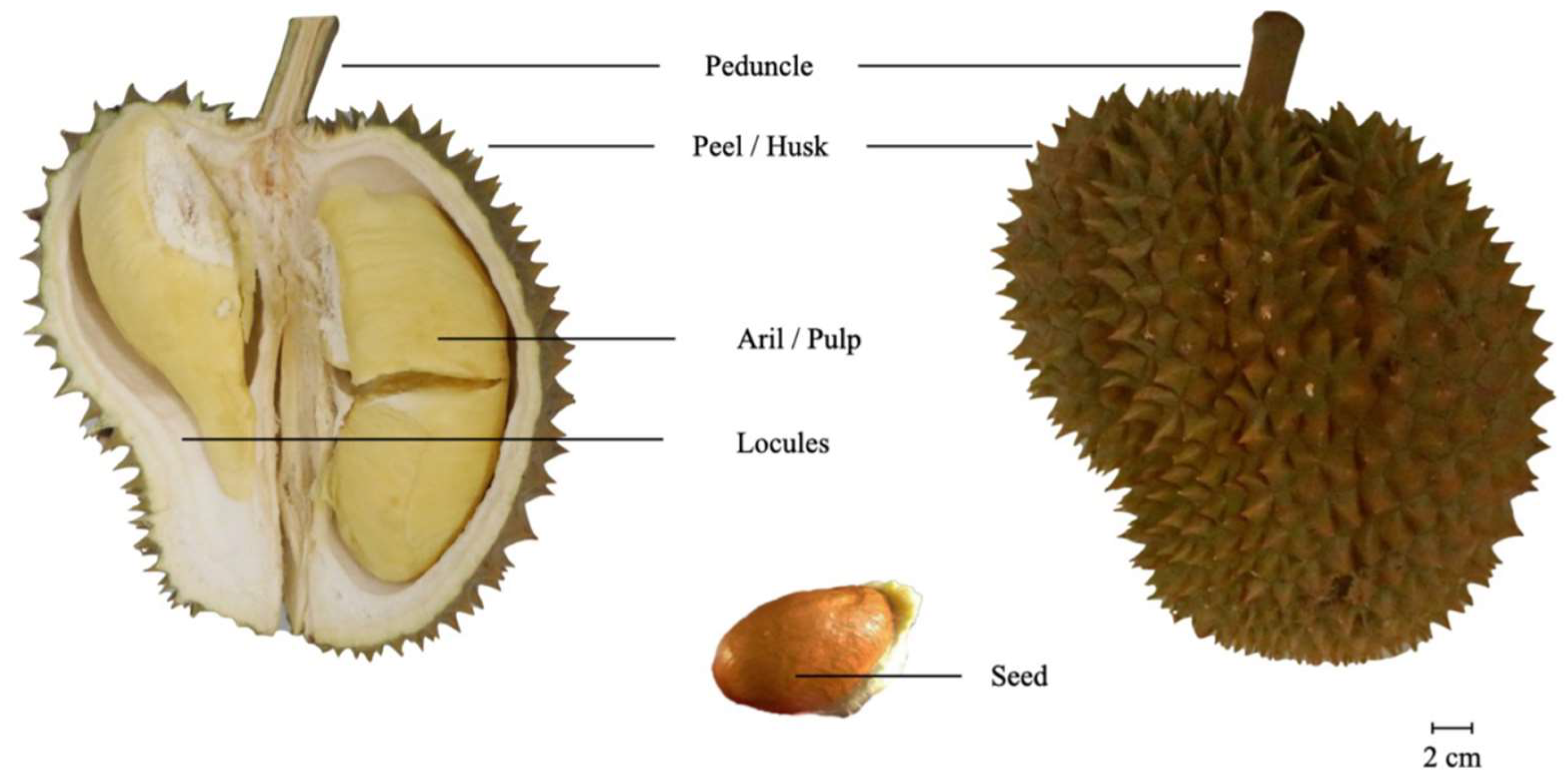The image is a detailed diagram of a durian, showcasing both its external and internal structures. On the right side of the illustration, an intact durian is depicted, while the left side reveals a cross-section of the fruit. The diagram is labeled with various parts: the top stem is labeled as "peduncle," indicating its connection to the tree. The outer surface, described as brown with small, pointy protrusions resembling triangles, is labeled "peel/husk." The internal section on the left shows a cream-colored "aerial/pulp" or "aril," with a white casing around it, designated as "locules." At the bottom of the image, a brown, bean-like seed is labeled as "seed." A scale in the bottom right corner indicates a measurement of approximately 2 cm.